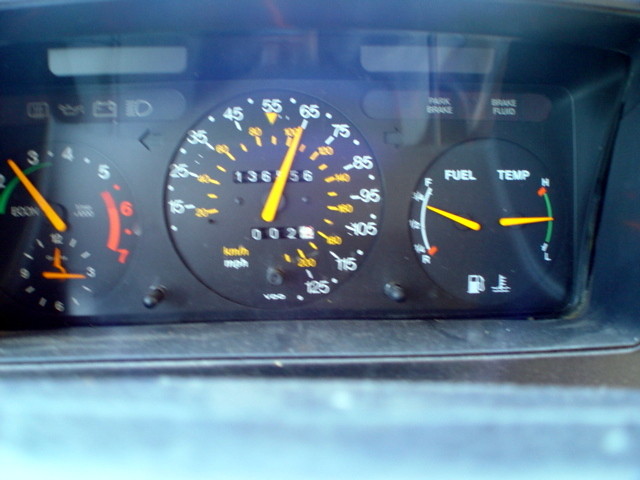The photo is a detailed close-up of a car dashboard, covered by a clear but noticeably dirty glass panel reflecting light, indicating it hasn't been cleaned for a while. On the left side of the dashboard, there's an instrument resembling a clock, marked with the numbers 12, 3, 6, and 9, and two hands. Above this, a section labeled 1 through 6 starts with green at 1 and transitions to red at 6, currently pointing between 2 and 3, possibly indicating engine temperature. Above this instrument are three icons: a square of indeterminate function, an engine light, and a battery light, accompanied by a symbol indicating headlights.

The central circle of the dashboard contains the speedometer, marked from 0 to 130 miles per hour, with an additional 5 miles per hour past 130. Inside the gauge, a section marked in yellow indicates kilometers per hour. The current speed is 65 miles per hour, and the car's odometer reads 136,556 miles.

To the right, a circular gauge labeled "Fuel" on the left and "Temp" on the right shows the fuel level at approximately three-fourths full. The temperature gauge indicates a level between low and high. Below these gauges, icons for gas and temperature are displayed.